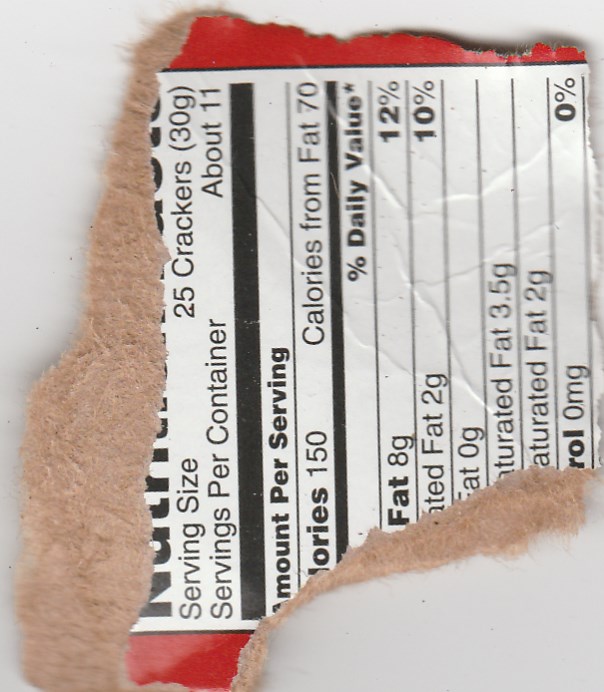This photograph captures a partially torn cardboard nutrition label of an unidentified food item. The image is rotated 90 degrees counterclockwise. Despite the tear, some details are visible, including a serving size of 25 crackers, which weighs 30 grams, and approximately 11 servings per container. The label indicates each serving provides 150 calories, with 70 calories from fat. Under the "% Daily Value*" section, it's partially legible that there are 8 grams of total fat, potentially 2 grams of saturated fat which is 12% of the daily value, and another kind of fat listed as 0 grams. Further details are obscured, but there's a potential mention of 3.5 grams of saturated fat and possibly 0 mg of cholesterol. The label features a white background, and the area around the torn section is slightly reddish, suggesting a tear effect.